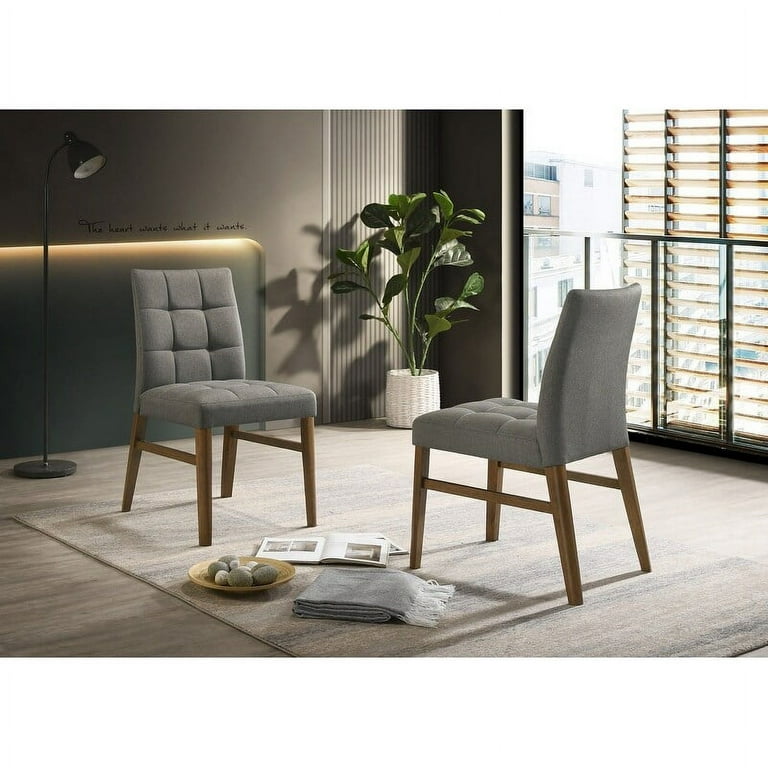This stock photo captures a modern and serene living area within a city apartment or condo unit. The room is illuminated by natural light streaming through a large window adorned with partially drawn blinds, offering a view of city buildings in the distance and casting dynamic shadows on the walls. Central to the image are two gray upholstered, armless chairs with wooden legs, positioned on a taupe and gray rug. Between the chairs, there is a beige, golden-hued plate filled with decorative gray and white spherical objects. 

A neatly folded gray blanket with white fringe and a couple of open books or magazines are thoughtfully arranged on the floor, adding to the room's cozy atmosphere. A tall, elegant black standing lamp provides ambient lighting, while a cursive inscription on the wall reads, "The heart wants what it wants," complementing the room’s aesthetic. 

In the corner, a lush green plant in a white basket or planter adds a touch of nature, its shadows enhancing the overall composition. The floor, featuring a wood grain pattern in taupe and gray hues, ties together the muted, modern color scheme of the space, which is dominated by pale blues, beige, and various shades of gray.